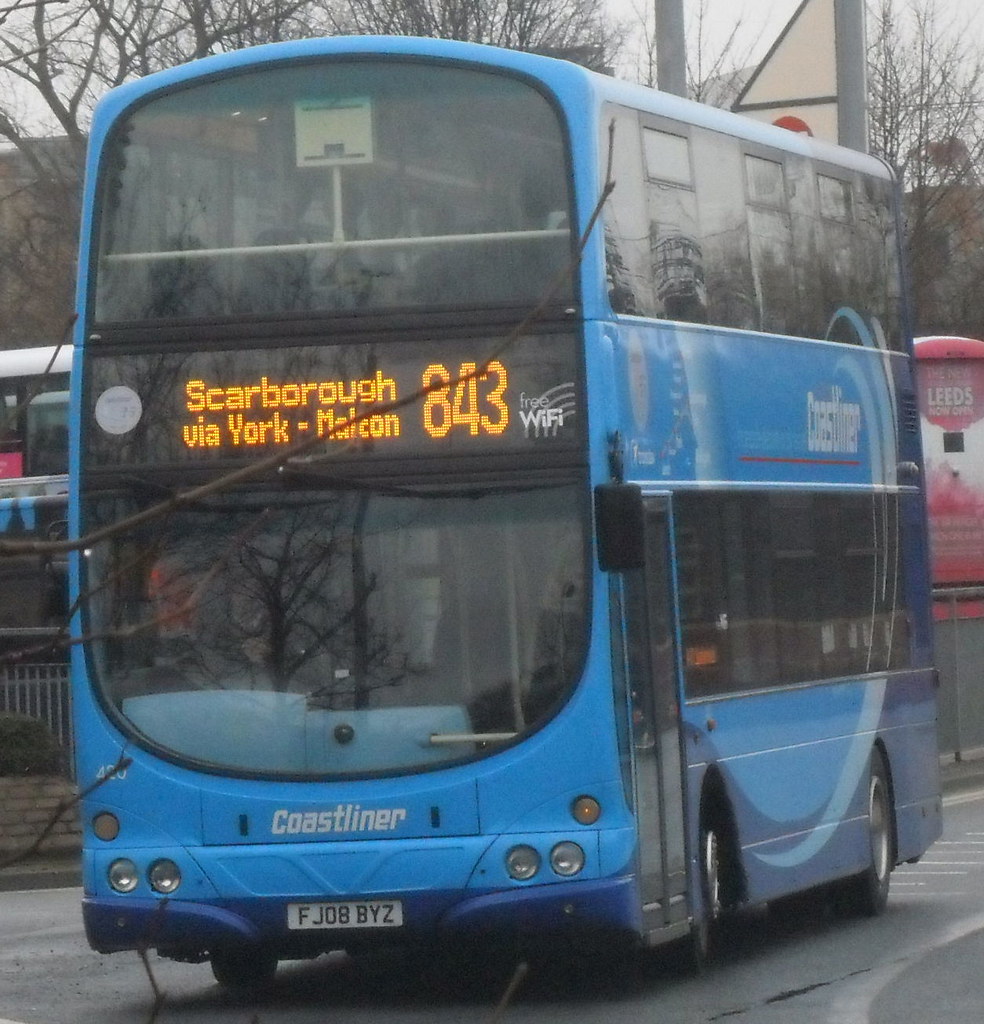In this detailed photograph, a light blue double-decker bus with dark blue accents is prominently featured, showcasing the company name "Coastliner" on its side. The bus is equipped with modern amenities, including free Wi-Fi, as indicated by a logo near the center. The front display, with bright orange text on an LED screen, announces the route "Scarborough via York, Malton 843." The bus is on the move, driving down a blacktop road, evidently during a fall or winter period, as indicated by the dry, leafless trees in the background.

Additional details include a glass panel that spans from top to bottom on the front of the bus, which also has two round headlights set low on the bumper and orange lights positioned above them. There is an accordion-style door at the front for boarding, and the exterior mirrors are encased in black housing. The bus also features large windows on both the lower and upper levels for passenger viewing. 

Partially visible in the background is another bus and a red sign that reads "The New Leeds Now Open." The license plate of the Coastliner bus is FJOB BYZ, and the scene also captures elements of a reddish vehicle amidst the landscape of barren trees, adding to the seasonal context of the image.